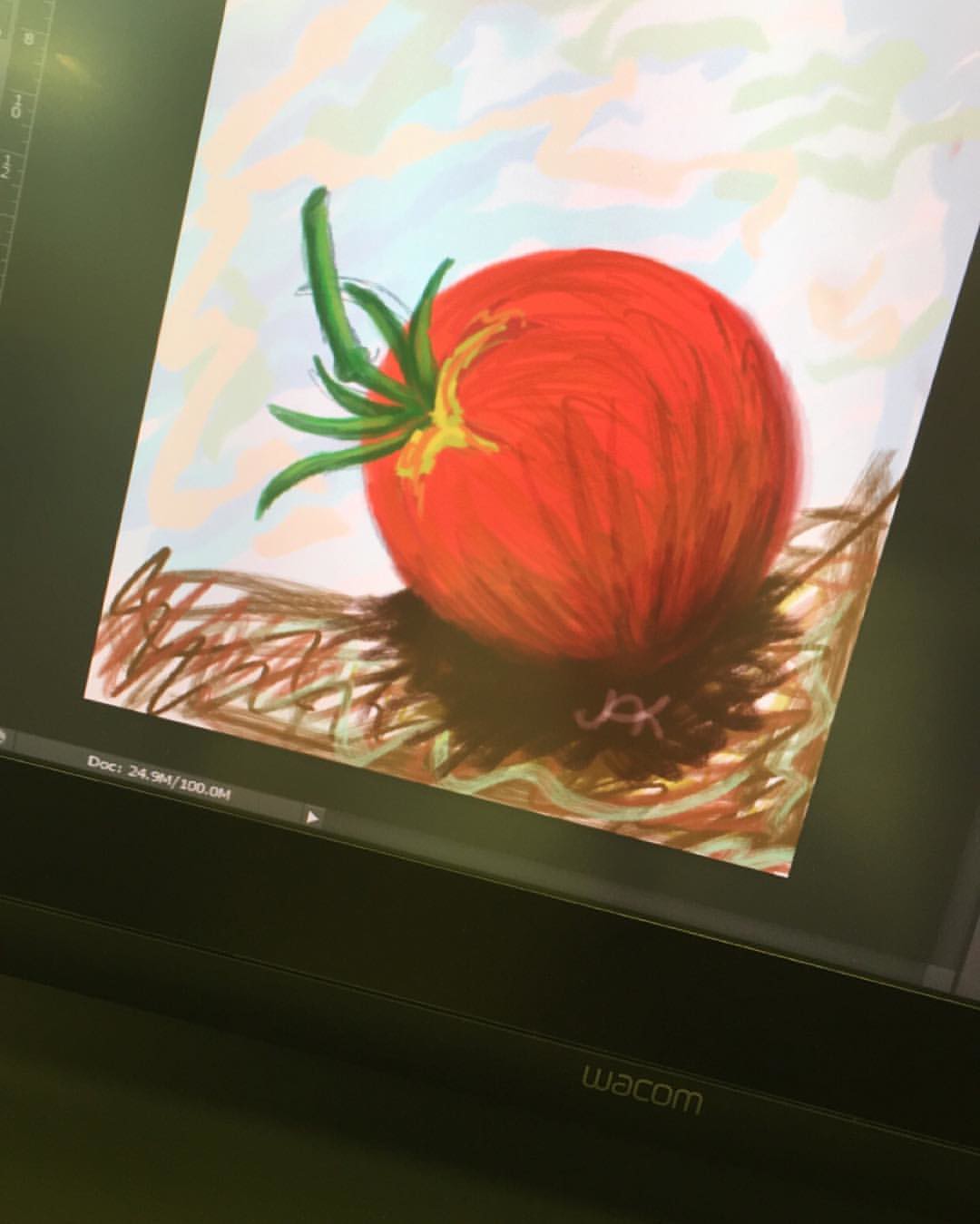A diagonally photographed computer screen displays an artistic drawing of a tomato resting on brown, squiggly-lined dirt. The tomato, lying on its side with its stem pointing left, is set against a backdrop of a blue sky adorned with clouds highlighted by white, gray, and light pink squiggly lines. In the bottom right corner of the drawing, the initials "JOK" are visible. At the bottom of the computer screen, informational text reads "DEC/DOC 24.9M / 100.DM" followed by an arrow. The brand logo "WACOM" is visible on the computer. The image is illuminated by a light source from the upper right side.